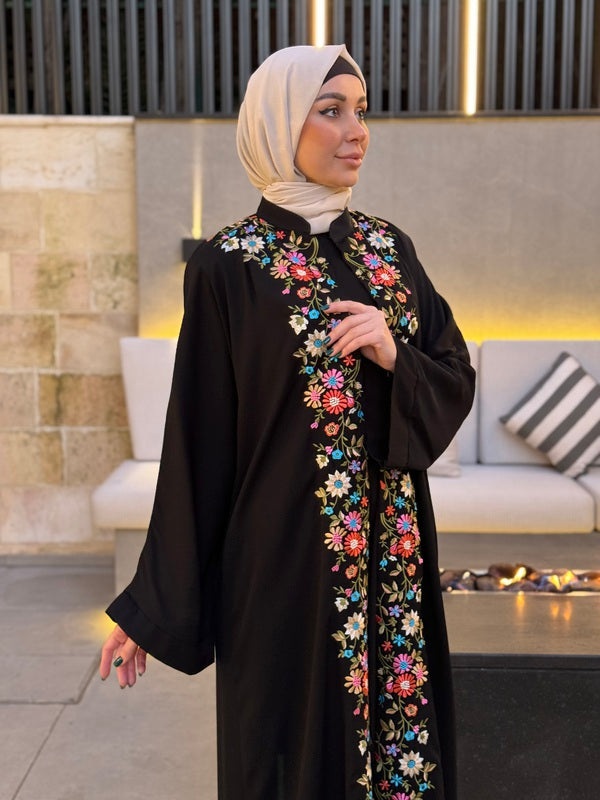This photograph captures a beautiful young woman standing in a portrait-oriented frame, dominating the height and length of the image. She wears formal attire—an elegant, black flowing robe adorned with intricately embroidered colorful flowers along the hemlines and collarbone. Her attire is complemented by a white hijab, underlaid by a black head covering that fully conceals her hair, and wrapped gracefully around her neck. Her nails are precisely manicured and painted a vibrant bluish-green. The soft, warm lighting bathes the indoor setting, emphasizing the rich and warm tones of her attire and enhancing the overall ambiance. Behind her, a softly focused sectional couch backs up against a well-lit wall, further illuminated by a sophisticated fire pit table. Adjacent to her on the left is a visible brick structure, adding texture to the background. She stands with poise, her left hand raised to her chest while her right hand rests lower, creating a balanced and serene posture that exudes grace and elegance. This meticulously composed image could easily serve as a high-quality editorial photograph, possibly highlighting the intricately embellished robe she is wearing.